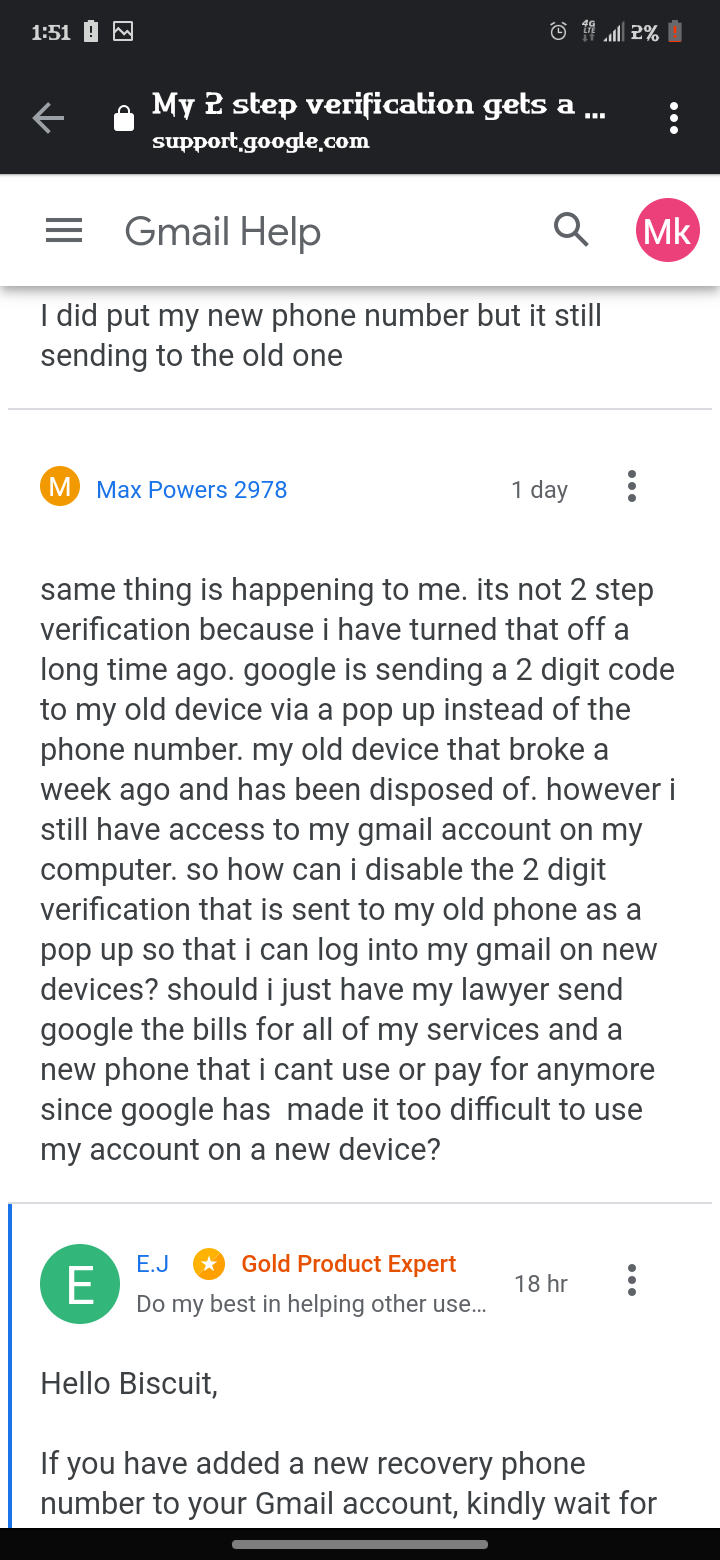Screenshot Description: Gmail Help Interface on a Smartphone

The image is a screenshot depicting a Gmail Help page on a smartphone. The time displayed in the upper left corner is 1:51. To the right of the time, there are several status icons: the first three icons include the alarm and Wi-Fi signals, followed by the cellular signal strength at 2%, and the battery icon. 

Directly below this, there is a row that includes a back arrow icon pointing to the left, a lock icon, and the text "My two-step verification gets a..." which is followed by an ellipsis. Beneath this header, the support.google.com URL is visible along with a menu icon.

The main header bar features a menu icon consisting of three horizontal lines stacked on top of each other. To its right, the text "Gmail Help" is displayed in bold with a capital "G". Further to the right, there is a search icon. Below this, the user icon appears as a pink circle with the letters "MK" in it, indicative of the user's initials.

The body of the page contains user-generated text stating, "I did put my new phone number but it’s still sending to the old one." This is followed by a reply marked by a yellow circle with the letters "MM" inside. The reply is from a user with the username "Max Powers 2978" in blue text, indicating they posted the reply one day ago. There are three vertical dots next to this comment, likely representing additional options. Below this, another comment is partially visible, marked by a green circle with the initial "E" inside.